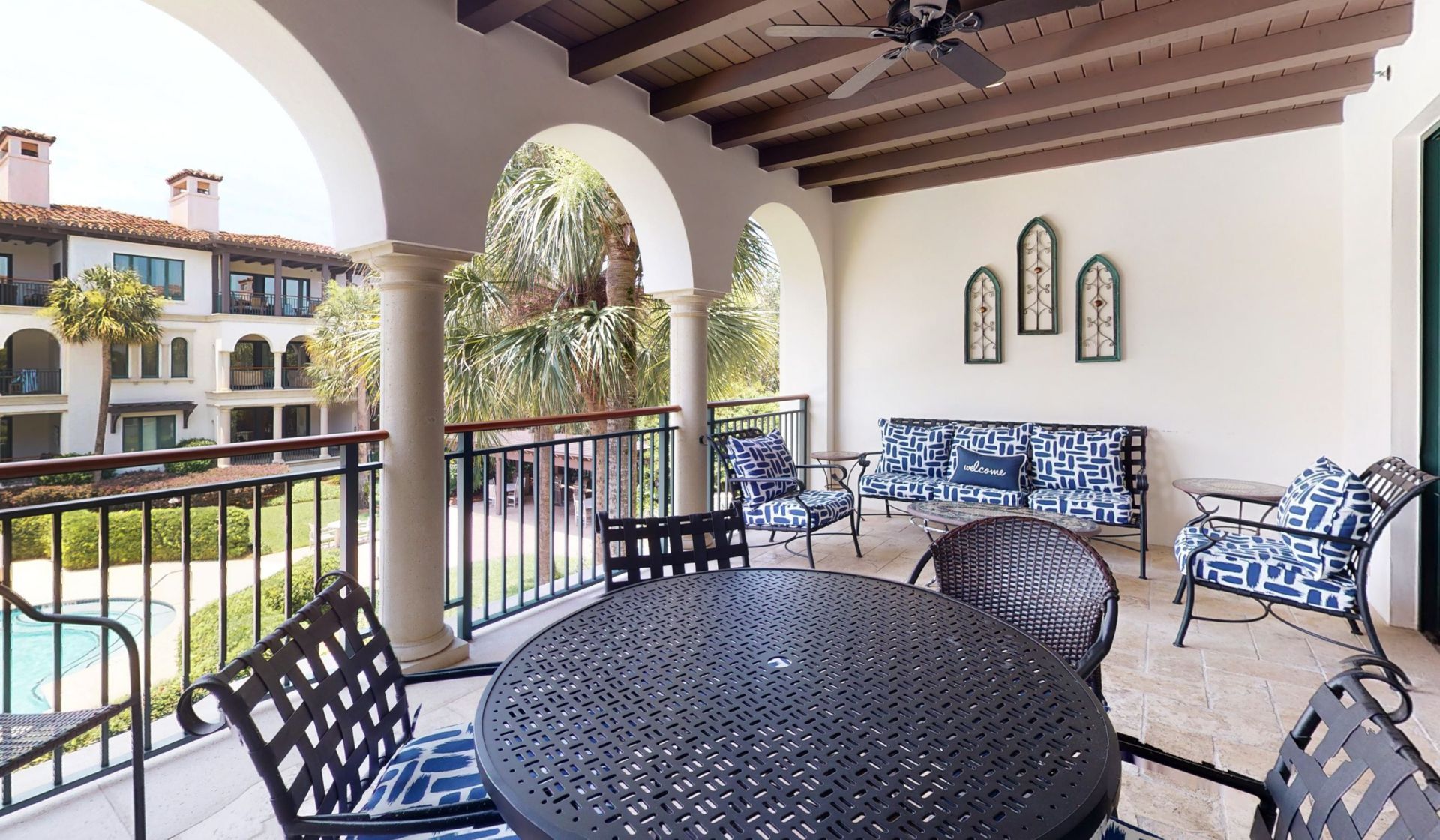The image captures an inviting outdoor patio at a resort, bathed in sunlight with sun rays beaming down on a serene, unoccupied setting. The patio overlooks a courtyard featuring a swimming pool framed by lush palm trees and green hedges. The patio is enclosed by a railing with vertical bars, punctuated by white pillars that support a roof with a wooden ceiling and an overhead ceiling fan.

The seating area is furnished with a round metal table surrounded by metallic chairs, each cushioned with blue and white striped fabric and featuring leather backings. One of the cushions bears a welcoming blue pillow. The floor of the patio is a light tan tile, enhancing the airy, comfortable atmosphere.

Against a white wall adorned with three wooden-framed wall hangings, there is a long bench seat with matching blue and white cushions, flanked by small chairs with the same cushion design. To the right, a doorway leads further inside the resort. Another building, identical to the one the patio is part of, is visible across the courtyard, reinforcing the resort's cohesive architectural charm. This picturesque scene epitomizes a luxurious and tranquil retreat.